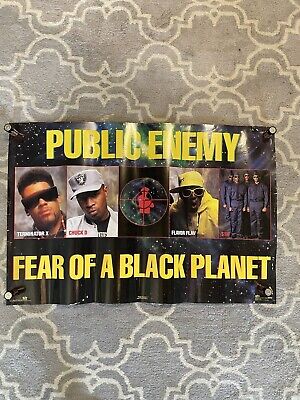The image depicts a rectangular poster set against a gray background adorned with horizontal, lantern-shaped white lines. The poster, which is seemingly held down at each corner by round, tall clips tipped in silver, prominently features the text "Public Enemy" at the top and "Fear of a Black Planet" at the bottom, both written in bold, yellow capital letters. The background of the poster is dark with scattered white dots. Centrally aligned, the poster showcases a horizontal series of five images: on the far left, a man with large black shades; next to him, another man wearing an Oakland Raiders hat; at the center, an image resembling the view through a rifle's sniper scope targeting someone; followed by Flavor Flav, distinguished by his all-yellow attire and shades; and on the far right, a group photo of four people in gray suits, with the poster resting on a rug beneath.